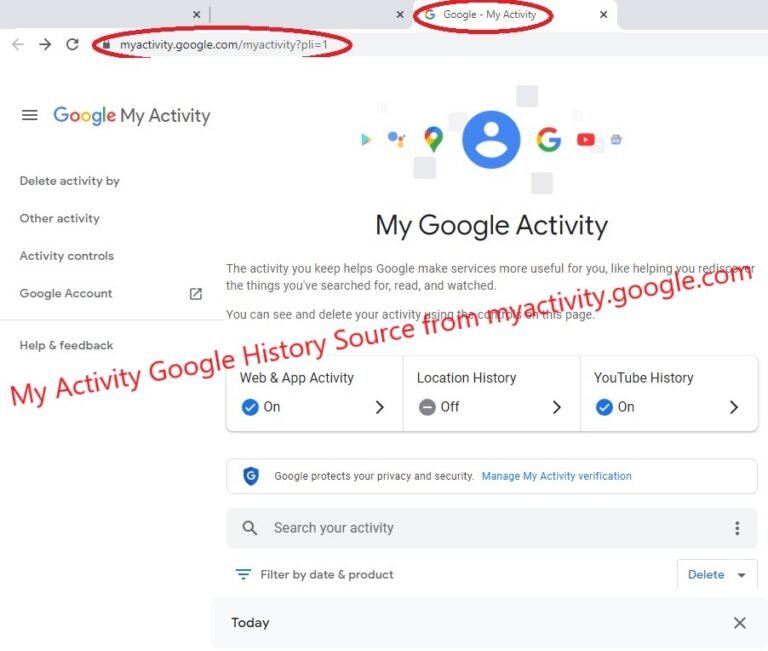**Screenshot of Google My Activity Dashboard: Detailed Description**

This screenshot captures the interface of Google My Activity, a subsection of Google where users can review their history of interactions across various Google services. In the top left corner, the interface prominently features the Google logo followed by the title "My Activity." 

On the left sidebar, a menu lists the following options: "Delete activity by," "Other activity," "Activity controls," "Google account," and "Help & Feedback." 

The main section of the page features a large title reading "My Activity," accompanied by a series of icons across the top representing different Google services. Starting from the left, these icons include:
1. Google Maps
2. An icon resembling a blue circle with a vertical yellow rectangle
3. Another Google service symbol, possibly the Google Play Store symbol
4. A generic person icon on a blue circle
5. The Google Search symbol
6. The YouTube symbol
7. An additional, unclear icon on the far right

Under the title, there are various activity controls that allow users to manage their web and app activity, YouTube history, and location history. These settings can be toggled on or off to personalize the activity tracking preferences.